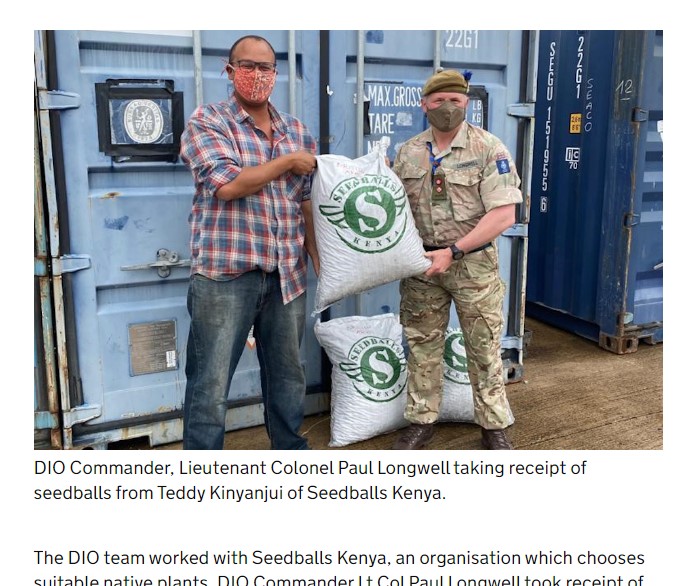This photograph captures two men in the process of handling large white sacks emblazoned with the logo of Seed Balls Kenya. The man on the left, with dark hair and dark-rimmed glasses, is wearing a red and white checkered surgical face mask, a blue, red, and white plaid shirt, and stone-washed blue jeans. His shirt is untucked on the left side and half-tucked on the right. He is holding the top of the white sack featuring a green circular logo with an 'S' and wings. Opposite him is a uniformed man dressed in khaki military fatigues and a beret, also masked. His attire includes a short-sleeved military-style shirt, camouflage pants tucked into brown boots, and he is grasping the bag's bottom edge. 

The scene is set against tall, blue metal locker doors with heavy hinges, and the ground beneath them appears to be dusty or dirty. Additional identical sacks of seed balls are placed at the feet of the military man. The caption at the bottom of the photograph reads: “DIO Commander Lieutenant Colonel Paul Longwell taking receipt of seed balls from Teddy Kinyanjui of Seed Balls Kenya.” It mentions briefly that the DIO team worked with Seed Balls Kenya to select suitable native plants, but the full description is cut off.